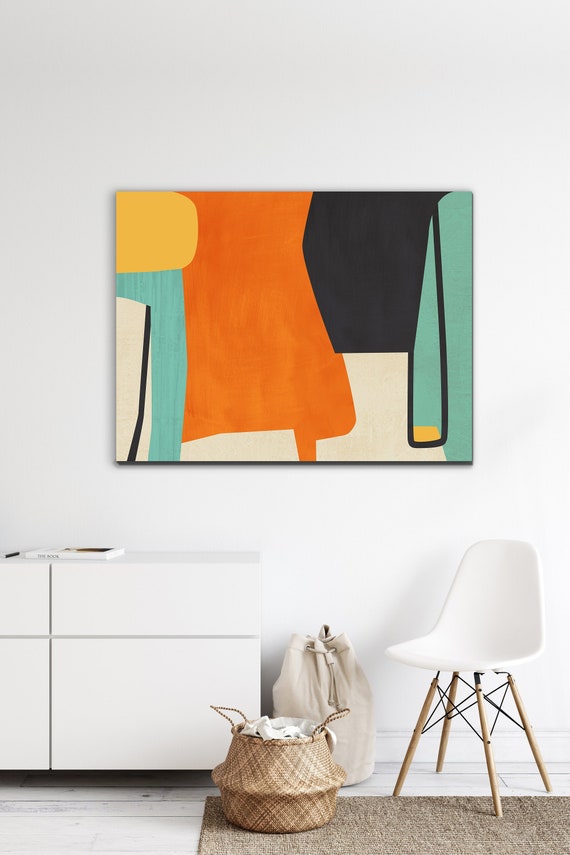The photograph captures a modern, minimalist apartment with white walls and white hardwood floors. Dominating the center of the image is an abstract painting featuring various shapes and vibrant colors, including yellow, orange, black, green, blue, and beige. Below the painting, a white dresser stands on the left, adorned with a book and a writing instrument on top. On the right, a contemporary white chair with wooden legs sits comfortably. Near the center of the floor is a beige knapsack and a brown, almost pot-like basket filled with white fabric, situated on a small brown rug. The clean, modern aesthetic is highlighted by the bright, tidy arrangement and the striking contrast of the colorful artwork against the otherwise monochromatic room.